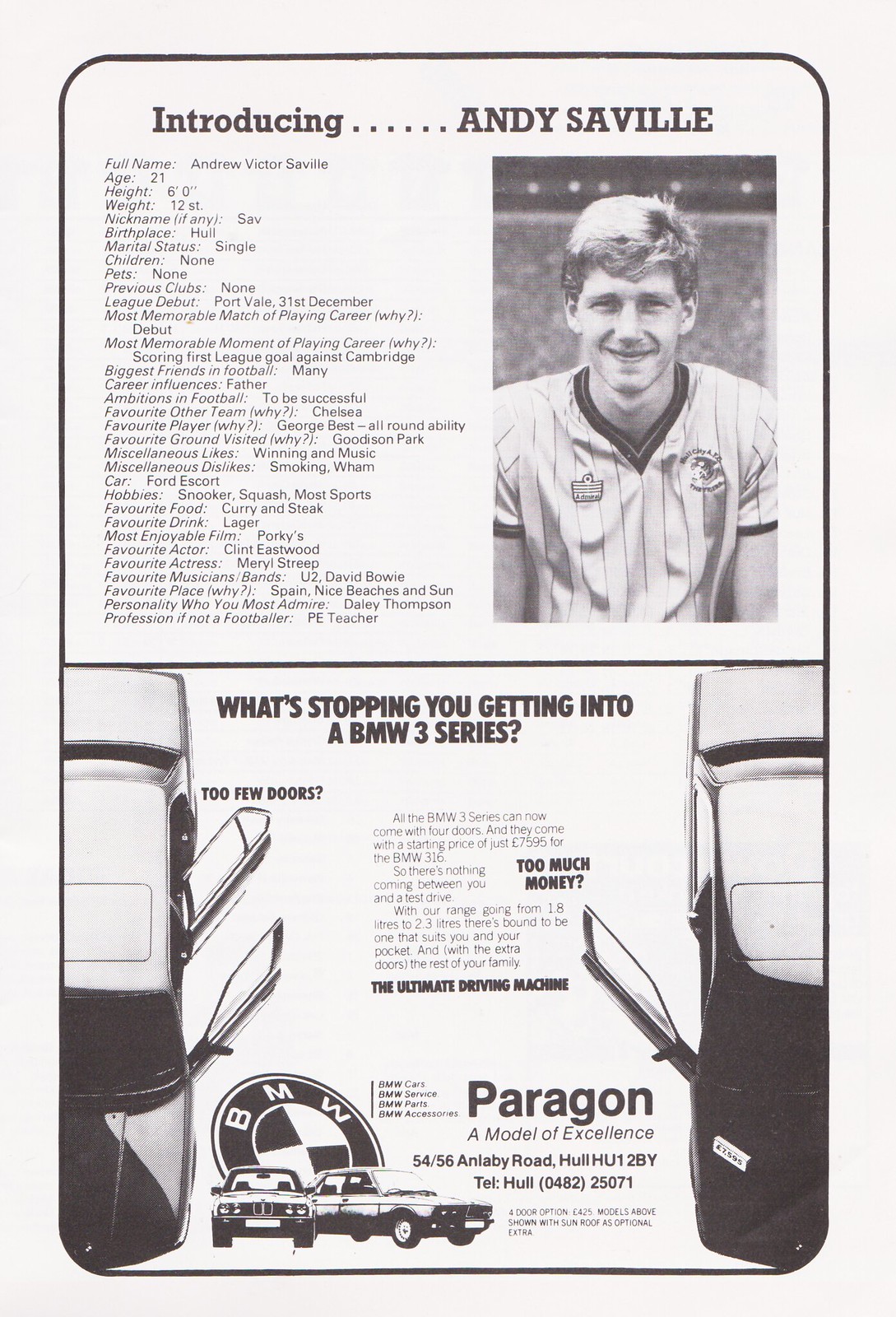The image displays a vintage page from an old sports magazine, divided into two sections. The top portion introduces Andy Saville, a young promising soccer player. His full name is Andrew Victor Saville. He is 21 years old, stands 6 feet tall, and weighs 12 stone. Known affectionately as "Sav," he hails from Hull. He is single with no children or pets. Andy has no previous club affiliations and made his league debut for Port Vale on the 31st of December. His most memorable career moment is his league debut and scoring his first goal against Cambridge. He admires George Best for his all-around ability, and his favorite team is Chelsea. His career ambition is to be successful in football, and he dreams of being a father. 

Outside of football, Andy enjoys playing snooker, squash, and other sports, with favorite activities including music and winning while disliking smoking and the band Wham. His favorite food is curry and steak, and his preferred drink is lager. "Porky's" is his most enjoyed film, Clint Eastwood and Meryl Streep are his favorite actors, and he admires musicians like U2 and David Bowie. He loves Spain for its nice beaches and sun. Andy looks up to Daley Thompson and, if not a footballer, he would have pursued a career as a PE teacher.

On the left of this section, the text is printed in a simple black font with a photo of Andy Saville on the right, wearing a striped shirt and smiling at the camera. The image is monochrome, and Andy appears to be of Caucasian descent with short hair.

The bottom section features an advertisement for BMW, displaying two cars with their doors open. Above the cars, the text reads, "What’s stopping you from getting into a BMW 3 Series?" On the left, the car is marked "too few doors," and on the right, it says "too much money." The ad highlights Paragon, a model of excellence, located at 5456 Anbleve Road, Hull, with the telephone number Hull 0482-25071. The entire page has an off-white, newspaper-like texture, with black and shades of gray dominating its color scheme. The layout is neatly bordered with a thin black stripe, giving it a classy, vintage feel representative of the early 1970s or 1980s era.